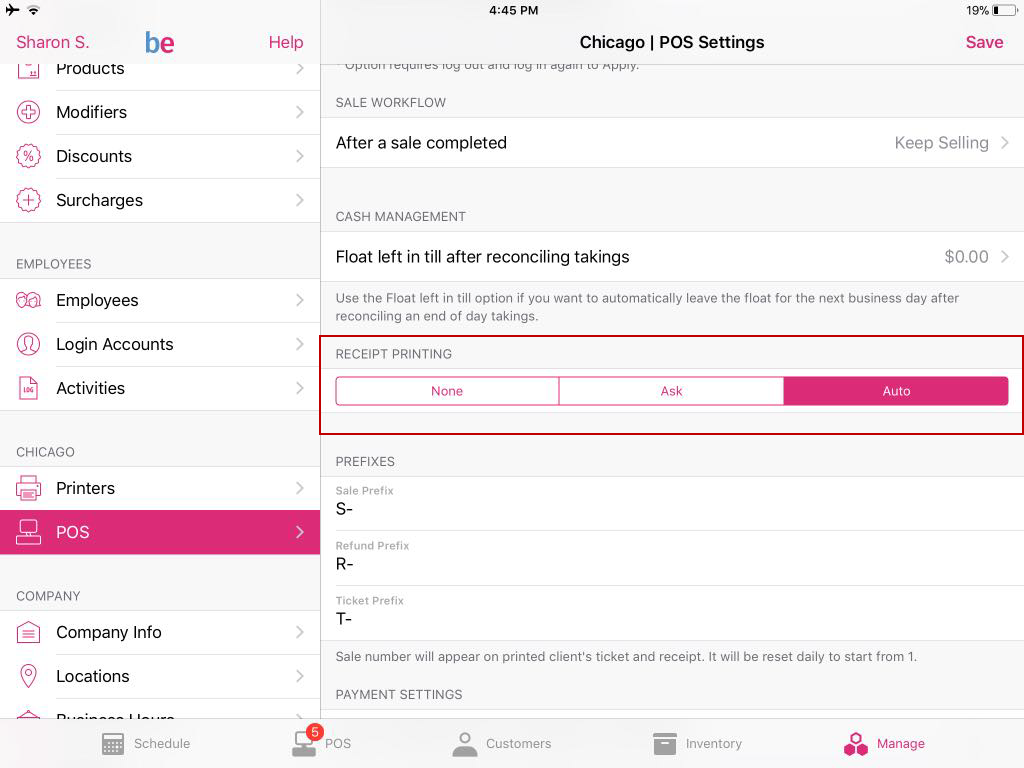Screenshot of Sharon S.B.E.'s website, likely named B.E., displaying comprehensive business management settings. The interface is divided into two main sections:

**Left Sidebar:**
- Lists various options:
  - Products
  - Modifiers
  - Discounts
  - Employees
  - Login Accounts
  - Activities
  - Printers
  - P.O.S. (Point of Sale)
  - Company Info
  - Locations
  - Business Hours

**Right Section:**
- Displays current time at 4:45 PM
- Battery level at 19%
- "Chicago P.O.S. Settings" headline
- "Sale Workflow" settings:
  - "After a sale completed, keep selling"
  - "Float left until after reconciling, taking zero dollars"
- "Receipt Printing" options: None, Ask, or Auto (highlighted with a box)
- Prefix settings:
  - Sales Prefix: S 
  - Refund Prefix: R 
  - Ticket Prefix: T 
- Statement indicating that the sale number will appear on the printed client's ticket and receipt, and will reset daily to start from one
- "Payment Settings" section listed below

The website appears to be a detailed application designed for managing sales and transactions in a business environment.